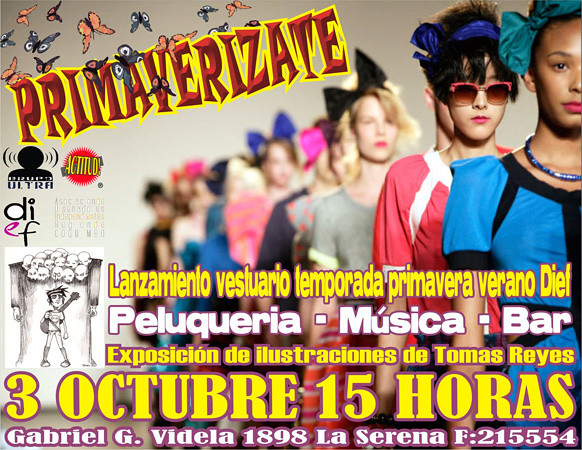This rectangular, horizontal advertisement showcases a lively and colorful scene. In the top left corner, bold red text with a yellow outline spells out "PRIMAVERIZATE," slightly angled with the right edge higher than the left. Scattered around the text are about ten vibrant cartoon butterflies in orange and blue. The main focus of the image features a line of diverse women in eccentric, brightly colored costumes, each adorned with a bow. The closest woman, partially cut off at the right edge, wears a blue dress with black trim and a green bow in her hair, complemented by a necklace. The second woman, donning red-framed sunglasses and a red dress, stands behind her. As the line extends backward, the women become increasingly blurred. The background is predominantly white, enhancing the vivid attire of the women. Below the image, in various colors and fonts, Spanish text reads: "LANZAMIENTO VESLUILARIO TEMPORADO PRIMAVERA VERANO D.L." In the middle, the words "MUSICA BAR" stand out in white, followed by additional text in bold yellow stating, "3 OCTUBRE 15 HORAS." The bottommost line provides further details: "GABRIEL G. VIDELA 1898 LA SERENA F. 215554."